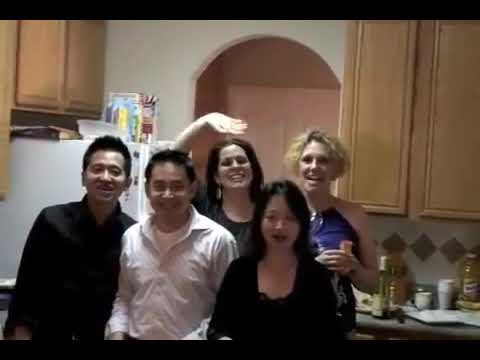The image depicts a group of five friends standing in a cozy kitchen, featuring beige cupboards, white walls, a refrigerator, and ample counter space with various kitchen supplies. In the front row, there are two Asian men and an Asian woman. The man on the far left is wearing a black button-up shirt, while the one next to him sports a white button-up shirt; both have short black hair and are smiling. The woman beside them, with long black hair, wears a black blouse and is also smiling. Behind them are two taller Caucasian women. The woman with long brown hair, wearing a green shirt, has her hand raised as if waving. The other woman, with short, curly, and frizzy blonde hair, is dressed in a blue dress and holds a wine glass. They all face the camera, aware of the photograph being taken, and their smiles suggest a warm, friendly atmosphere. The kitchen's left side shows a white refrigerator, while the right side reveals more wooden cabinets and counter space filled with bottles and cups. The photo captures a joyful moment among friends in an indoor setting, likely taken during a casual gathering.